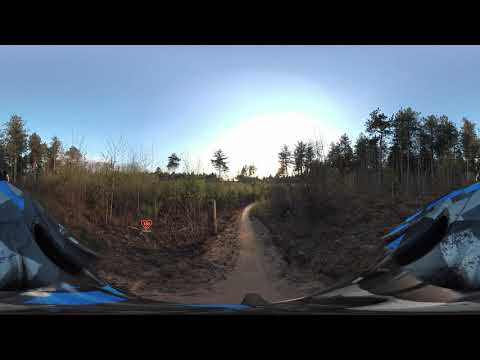The image captures an outdoor scene, showcasing a dirt pathway framed by dense, green trees and native plants. The path, a mix of brown earth and small rocks, descends slightly, suggesting an off-roading adventure. The photograph seems to be taken from a motorcycle or similar recreational vehicle, partially visible at the bottom of the frame with a blue front and possibly a windshield reflecting the bright sunlight. The sky above is a clear, vibrant blue, free of clouds, enhancing the picturesque midday setting. An official brown sign with gold lettering stands along the path, hinting at the natural area's significance. The overall composition, marked by natural elements and vivid colors, immerses the viewer in a serene, adventurous outdoor experience.